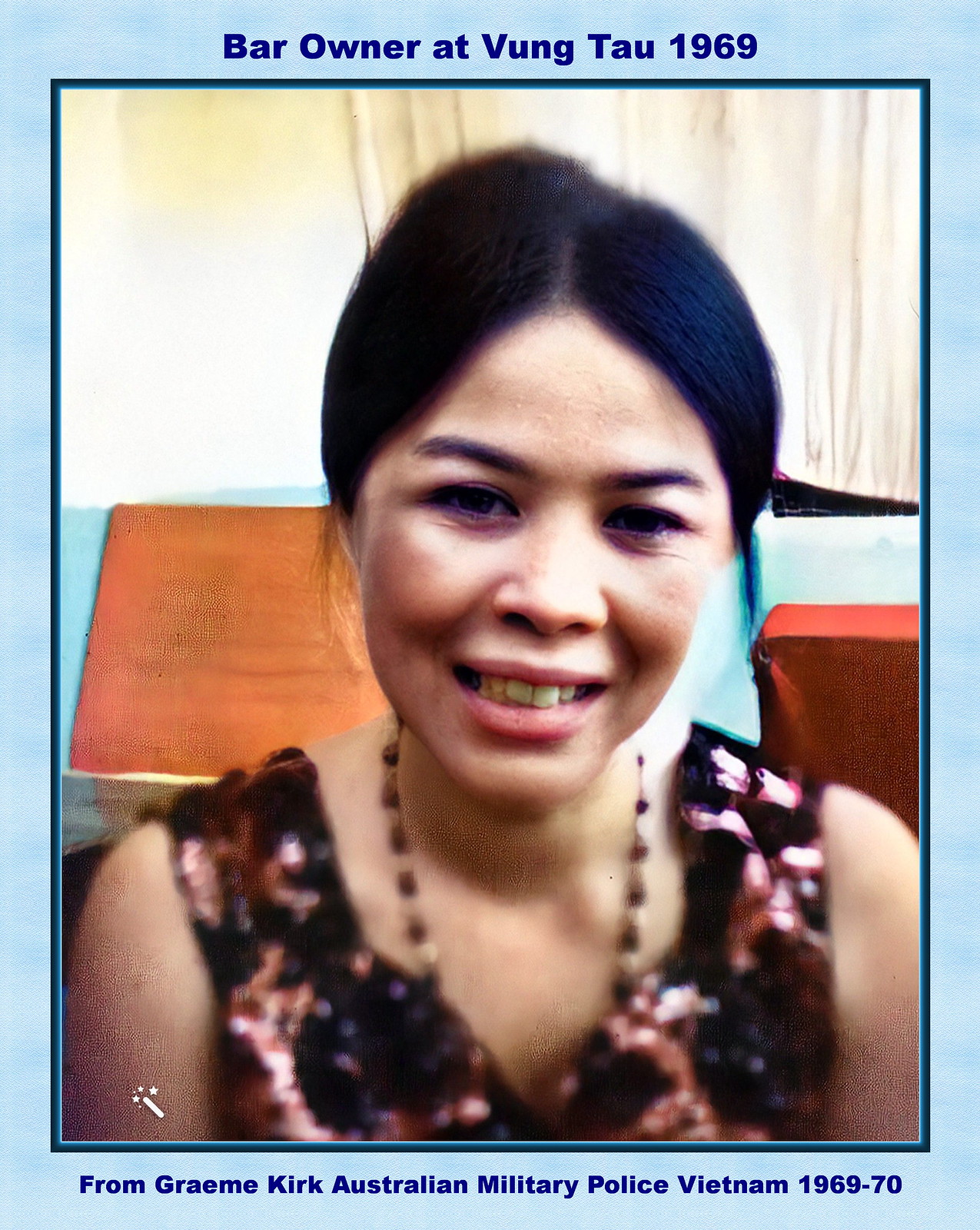The image features a color photograph from 1969 of an Asian woman, assumed to be Vietnamese, surrounded by a light and dark blue border, reminiscent of a baseball card format. At the top of the image, blue lettering reads "Bar owner at Vung Tau 1969," and at the bottom, it says "From Graham Kirk, Australian Military Police, Vietnam, 1969-70." The woman, smiling with her head slightly tilted, has dark hair pulled back and is wearing a floral tank top in dark colors, along with a bead necklace. Her exposed arms and chest are visible, and behind her, indistinct curtains and possible furniture can be seen. The photograph, slightly blurry, raises curiosity about its connection to the Australian Military Police and the woman's story during that period.